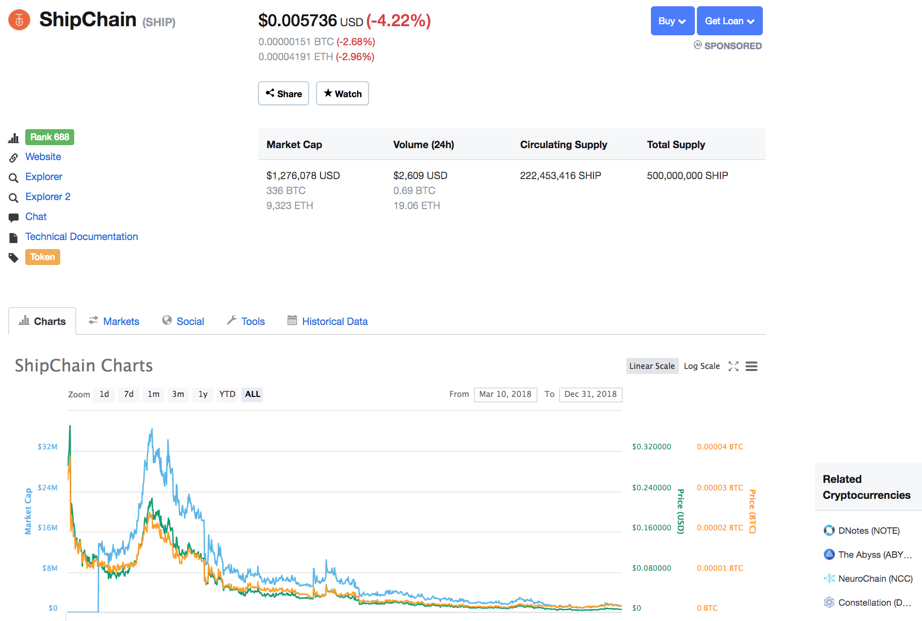This screenshot appears to depict a cryptocurrency monitoring interface on a computer screen, although it is unclear whether it is from a website or a standalone software application. The background is a solid white. In the top-left corner, an orange icon featuring a white design sits beside bold black text reading "Ship Chain," followed by "SHIP" in gray within parentheses.

On the upper-right corner of the interface, there are two blue horizontal buttons with white text. The button on the left reads "Buy" accompanied by a downward arrow, while the button on the right says "Get Loan" with a downward arrow beneath. Below this second button, the term "Sponsored" appears in light gray text.

Centrally located on the screen is the price "$0.005736 USD" displayed prominently, with "-4.22%" in red parentheses indicating a price decrease. Below this, there are additional statistics related to Bitcoin (BTC) and Ethereum, identifying key financial metrics. Underneath these details are two white buttons outlined in gray: one labeled "Share" in black text and the other "Watch."

On the left-hand side, a vertical series of hyperlinks is displayed. The top link is enclosed in a green button with white text that reads "Rank 688." Below this, there are blue hyperlinks for "Website," "Explorer," "Explorer 2," "Chat," "Technical Documentation," and an orange button at the bottom with white text that reads "Token."

The right-hand side of the screen features a gray bar divided into four labels: "Market Cap," "Volume," "Circulating Supply," and "Total Supply," each with corresponding financial figures displayed beneath.

At the bottom of the interface, a graph chart is visible. At the top-left of this chart are five tabs. The first tab, labeled "Charts" and illustrated with a bar graph icon, is selected in black. To its right, four more blue-labeled tabs include "Markets" (with a diagonal gray line), "Social" (with a globe icon), "Tools" (with a gray wrench), and "Historical Data" (with a gray calendar). The header below reads "Ship Chain Charts," surrounded by gray labels for various graph options, including "Zoom," "1 Year," "Year to Date," and "All," alongside date filters set from March 10, 2018, to December 31, 2018. Graph settings options like "Linear Scale" and "Log Scale" appear to the right.

The graph itself contains green, yellow, and blue lines representing different performance metrics, with green at the lowest, yellow in the middle, and blue performing the best. The vertical axis on the left is labeled "Market Cap," while the right side shows "Price USD" in green, alongside a series of prices. An additional column of information in orange color displays the "Price BTC."

Finally, at the bottom right, there’s a gray bar labeled "Related Cryptocurrencies" in black text, listing four names underneath: "D Notes," "The Abyss," "NeuroChain," and "Constellation."

This detailed, organized interface provides an extensive array of financial and market data for cryptocurrency tracking and analysis.